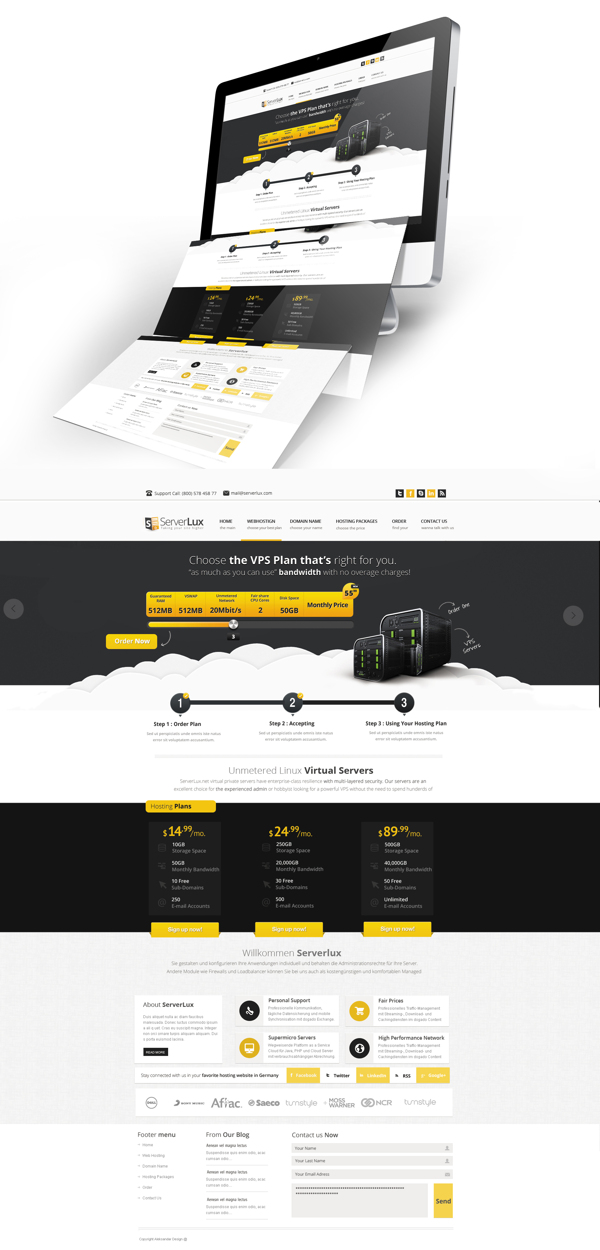The image depicts a vibrant, well-designed section of Serverlux's website, dedicated to showcasing various VPS (Virtual Private Server) plans. The color scheme predominantly features sleek black and vibrant yellow, creating a modern and engaging appearance. 

At the top of the screen, a computer monitor displays the same website, seemingly printing out its contents repetitively, adding a dynamic, tech-savvy touch to the overall design. The main content is set against a background of soft, whimsical clouds, making the page visually appealing and easy to navigate.

Serverlux offers a clear, three-step plan to help users select the VPS package best suited to their needs, with three tier options: $14.99, $24.99, and $89.99. These plans are designed to cater to a range of requirements and budgets, with emphasis on generous, overcharge-free bandwidth usage.

The website is dotted with numerous testimonials, emphasizing high customer satisfaction and reliability. At the top left corner, the Serverlux logo is prominently displayed, reinforcing the brand identity. The website also features endorsements from well-known partner companies, enhancing credibility and establishing Serverlux as a respected player in the virtual server industry.